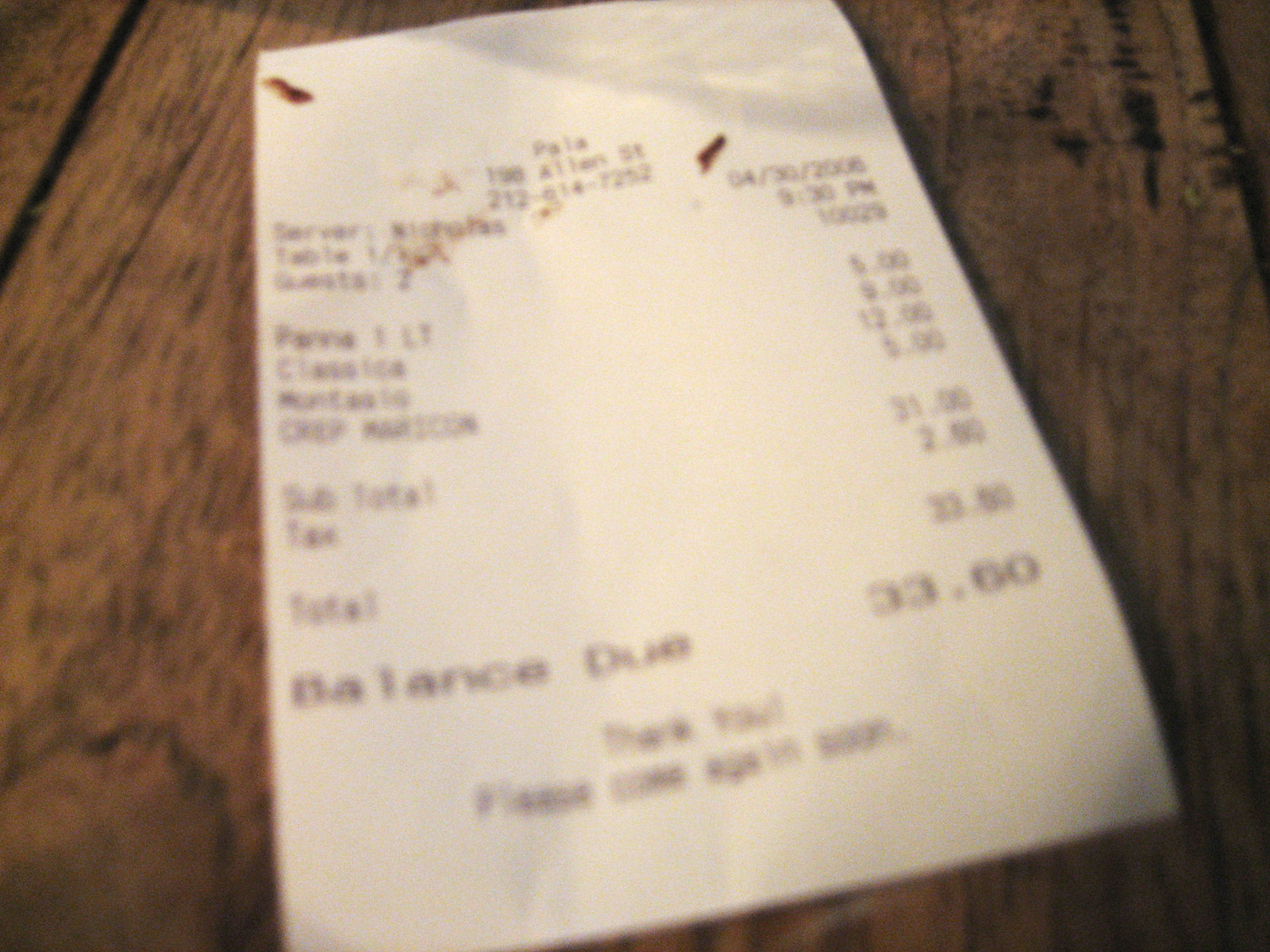In the photograph, a slightly blurry white receipt is placed predominantly over a wooden table. The table features visible brown planks arranged vertically, with a distinct grain pattern that has darkened patches, adding depth and texture to its surface. The receipt, angled slightly to the right, is legible enough to identify that it originates from a place named "Pala," suggesting it is from a restaurant. Notably, the bottom of the receipt states a balance due of $33.60, followed by a courteous message: "Thank you, please come again soon." The receipt appears slightly soiled, with small brown specks suggestive of food stains scattered across it. These marks are more concentrated near the upper left corner and right side, possibly indicating that someone with food residue on their hands handled the receipt. This detail contributes to the authenticity of the dining experience captured in the image.